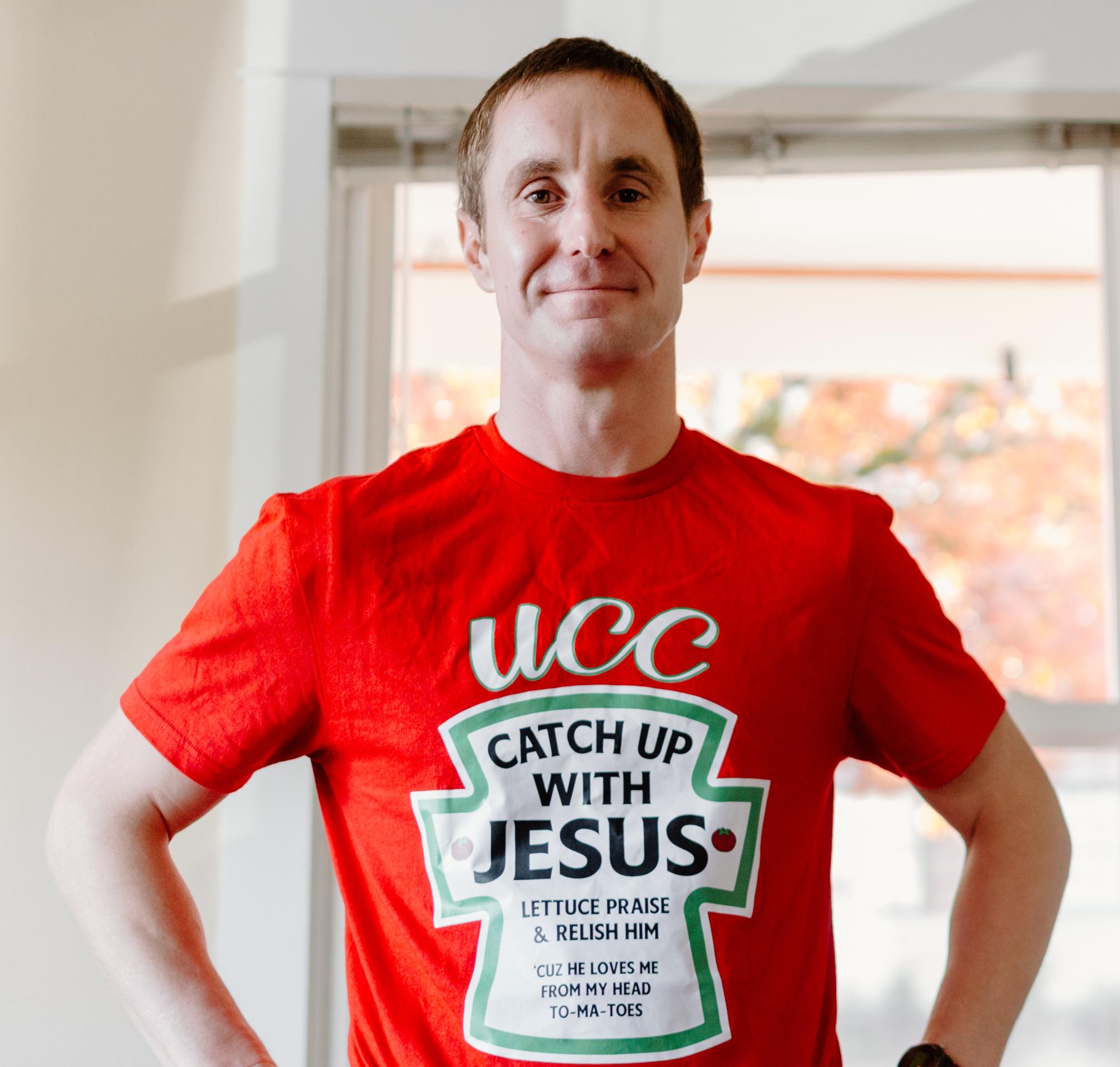In the image, a man with short brown hair stands with his hands on his hips, exuding a half-smile or perhaps a pursed-lip expression. He is positioned against a light tan wall with a window behind him, through which orange-colored trees are visible. The window features a white frame that contrasts softly with the background. The man is wearing a bright red t-shirt adorned with a playful design resembling the iconic Heinz ketchup label. The shirt features the letters "UCC" at the top, surrounded by a green outline, resembling cursive white lettering. Below it, a cross with a green inset border has text inside that whimsically reads "Catch Up with Jesus." Further down, the shirt continues with the message, "Lettuce Praise and Relish Him," followed by "Because He Loves Me from My Head to My Toes." The clever wordplay incorporates elements like "catch up" and "lettuce" to resemble "ketchup" and "lettuce," adding to the humorous and thoughtful theme of the shirt. The man is also sporting a watch on his left wrist, completing his casual yet distinctive look.